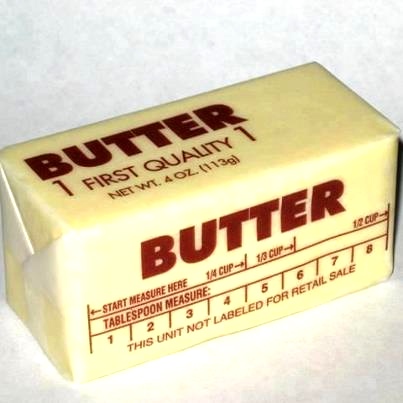This image features a stick of butter wrapped in white paper, placed at a roughly 40-degree angle against a whitish-gray background. The butter itself is a golden yellow color. The top of the packaging prominently displays "BUTTER" in large, dark brown block letters, followed by smaller text reading "First Quality" and "Net Weight 4 oz (113 g)." Along the side of the stick, “BUTTER” is written in maroon letters accompanied by a detailed measuring guide ranging from one to eight tablespoons. The guide provides measurements in tablespoons and cup fractions, specifically a quarter cup, a third of a cup, and half a cup. Additionally, it notes, "This unit not labeled for retail sale."